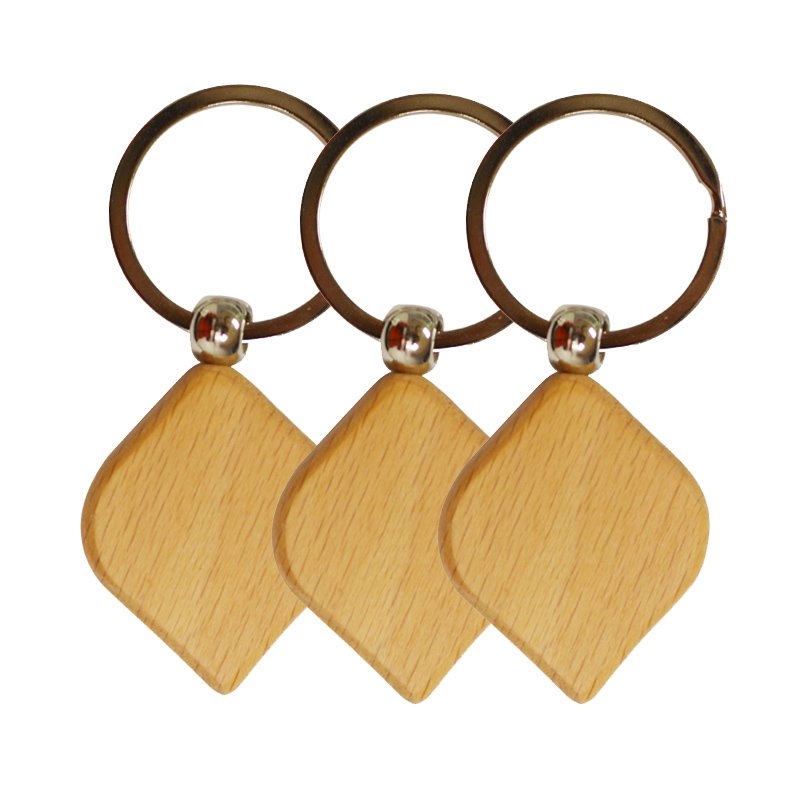The image depicts three identical objects arranged against a completely white background. Each object consists of three main components. At the top, there is a round, dark brown, metal ring that resembles a keychain. This ring is connected to a shiny, steel-like, silver connector. Below the connector is a wooden piece with a light, blonde hue, shaped in a way reminiscent of a square with rounded edges, tapering into a twisted, teardrop-like form. The wooden part is described as looking similar to a cutting board or even a slice of toast, which hangs from the bottom, giving an impression of two triangular shapes connected at their tips. The rings overlap from left to right, presenting an illusion of a singular unit rather than individual pieces. The precise function of these objects remains unclear, as they could be keychains, earrings, or another form of jewelry.